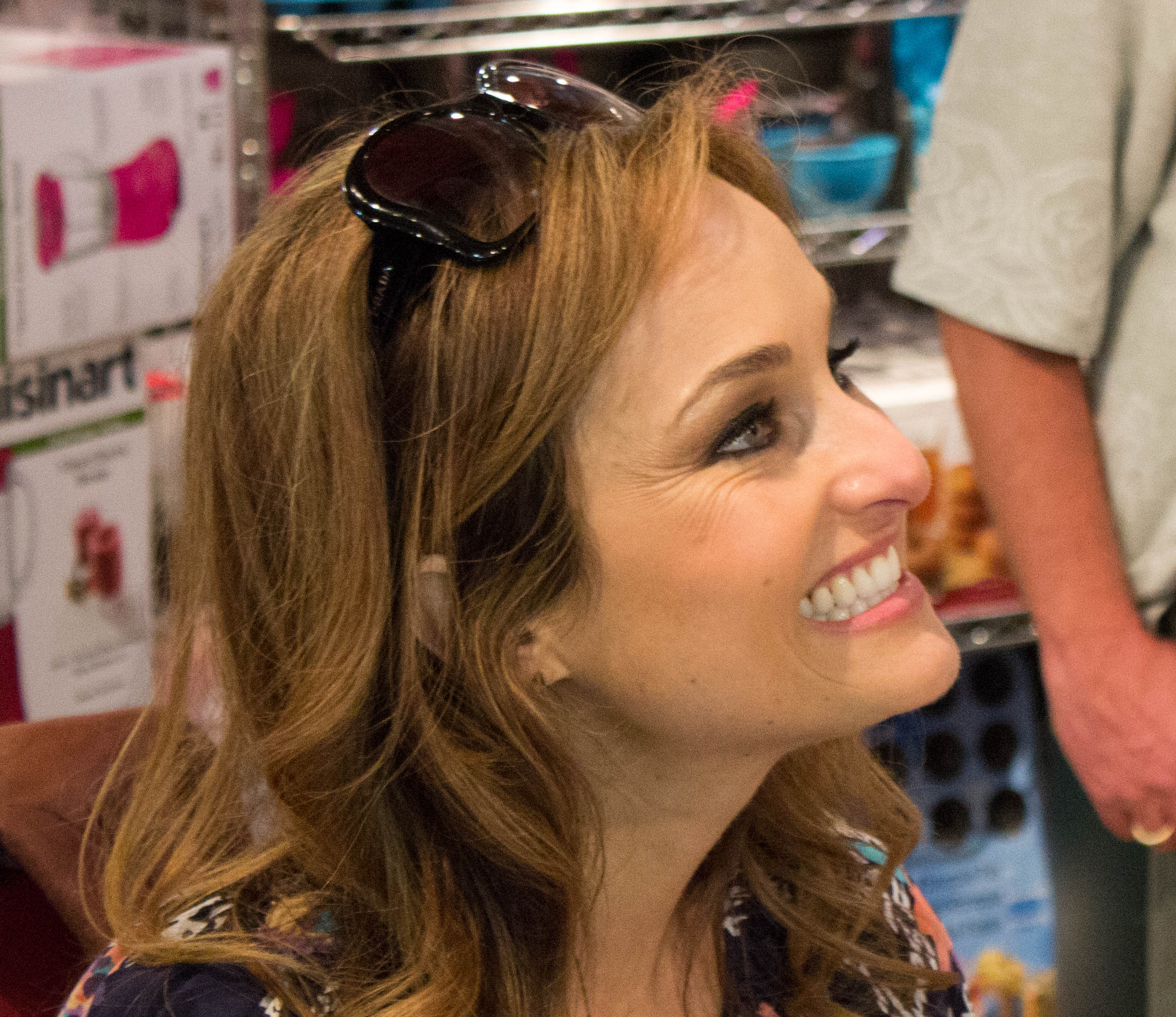The photograph captures a woman with shoulder-length dirty blonde hair, adorned with large, square-shaped black sunglasses resting on top of her head. She is facing slightly to the right and looking upwards with a smile that appears somewhat forced and unnatural. Her complexion is heavily made-up, featuring thick eye shadow, very pink lipstick, and perfectly white teeth. She dons a black top decorated with various colored patterns, though the exact design is difficult to discern due to the photo's angle. Behind her, wire shelves display various kitchen appliances, including a box featuring a bright pink blender. To the right of the woman, partially cropped out, stands a person in a short-sleeved gray shirt with a ring on their finger, indicating they might be male. The setting appears to be a store that sells these types of household items.